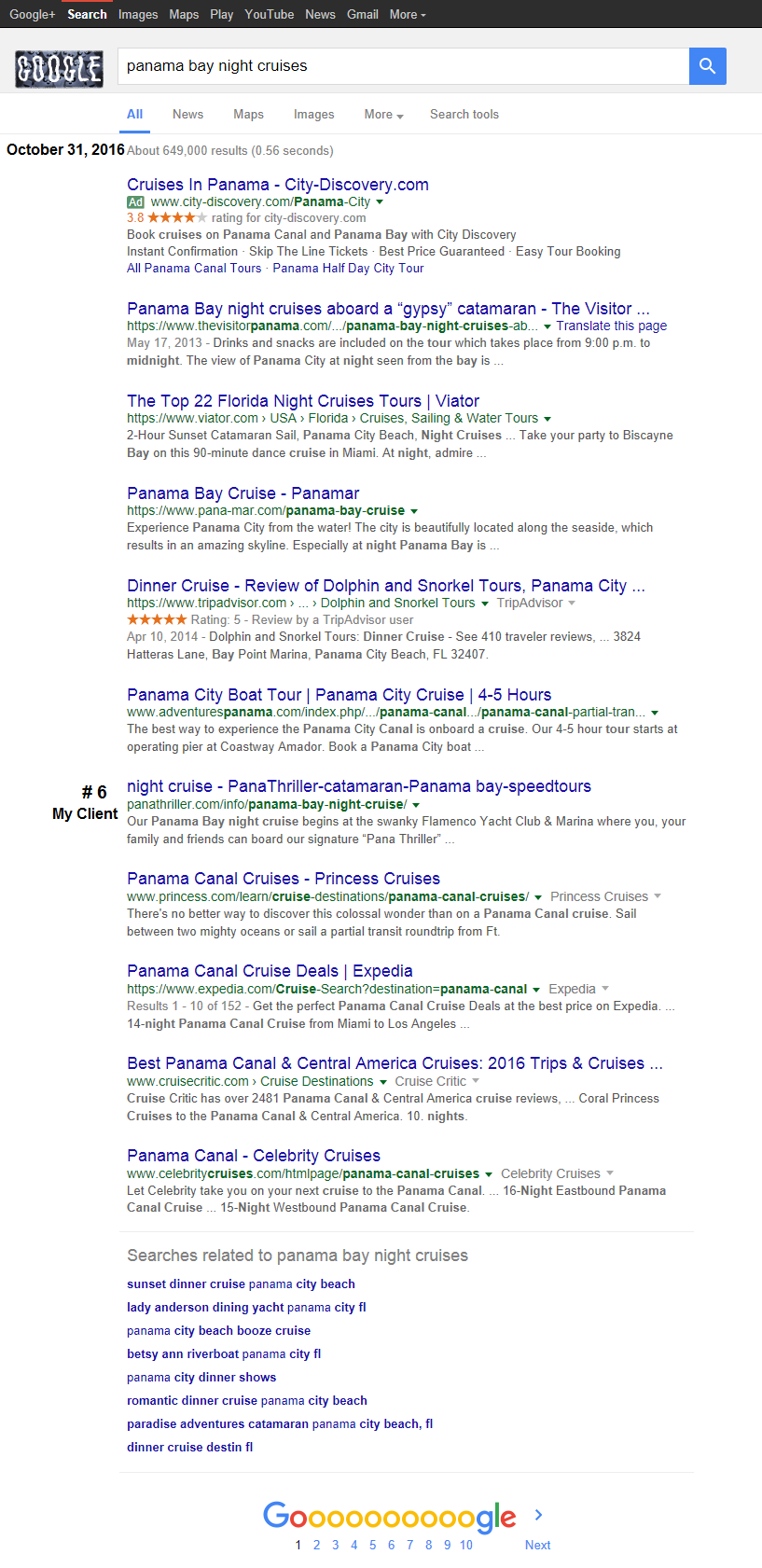Screenshot of a Google search conducted on October 31, 2016, displaying Google's classic white background layout. The search query entered is "Panama Bay night cruises," yielding approximately 649,000 results in just 0.56 seconds. This is a scrolling screenshot, spanning about two to two-and-a-half times the vertical length of a typical tablet screen.

The search results include various listings, with the first being a sponsored ad from cruisesinpanamacity-discovery.com. Underneath the ad, there are six organic search results. Notably, the sixth result is marked in the left margin with a text in black reading "number six, my client." This specific result is a link to Night Cruise, Panathriller, Catamaran, Panama Bay Speed Tours from panathriller.com, indicating a successful SEO effort to achieve a top placement.

Following these results, there are four additional listings visible before reaching the end of the first page of the search results. At the bottom of the screenshot, suggestions for similar searches related to "Panama Bay night cruises" are shown, along with the iconic Google logo. Beneath each letter in "Google," the page numbers 1 through 10 are listed, highlighting that the viewer is currently on page one.